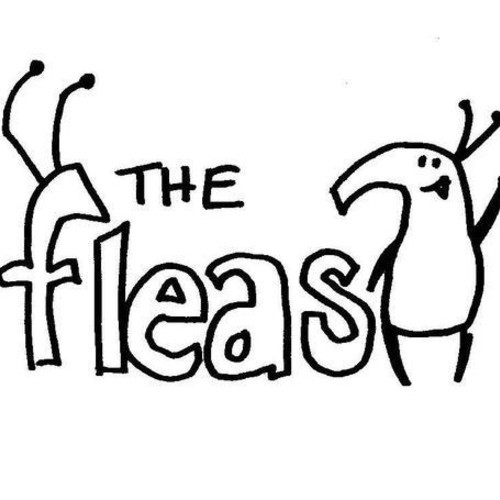The image features a hand-drawn or digitally created cartoon icon set against a stark white background. Central to the design is the bold, block-lettered text "The Fleas." Above the word "Fleas," the article "The" is written in a smaller size. The letter "F" in "Fleas" has two antenna-like extensions with small black dots at their tips. Adjacent to the text, near the letter "S," stands a whimsical character resembling a flea or bug. This anthropomorphic figure, standing upright on two stick-like legs, has a smiling face and raises one of its stick arms in a friendly wave. The entire composition is simple yet charming, suggestive of a child's drawing or a primitive cartoonist's style, possibly intended as a playful art project or logo.